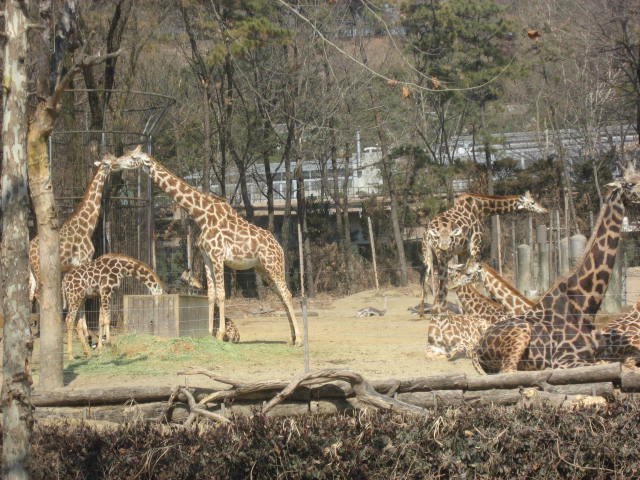This detailed image captures a vibrant giraffe enclosure at a zoo, with several giraffes of varying sizes and spot patterns. The scene is lively with a mix of giraffes standing and sitting, some resting in the shade while others interact with their environment. On the left side, two giraffes appear to be staring directly at each other, creating a moment that looks almost like a kiss from this perspective. Another giraffe nearby bends its neck to eat from a wooden box, with yet another sitting in the shade in front of it. Moving to the right, there's a giraffe bent down, seemingly curious about something on the ground, while more giraffes rest comfortably. Enclosing this animated scene is a wooden fence backed by chicken wire, with dark green shrubbery lining the front. The ground inside the enclosure features green-yellow patches of grass and several tall, thin trees—some bare, some with green leaves—adding a natural look to the setting. In addition to the greenery, there are wooden logs in the foreground and another taller cylindrical cage structure to the left. This serene daytime image vividly showcases the varied behaviors and interactions of giraffes within their zoo habitat.